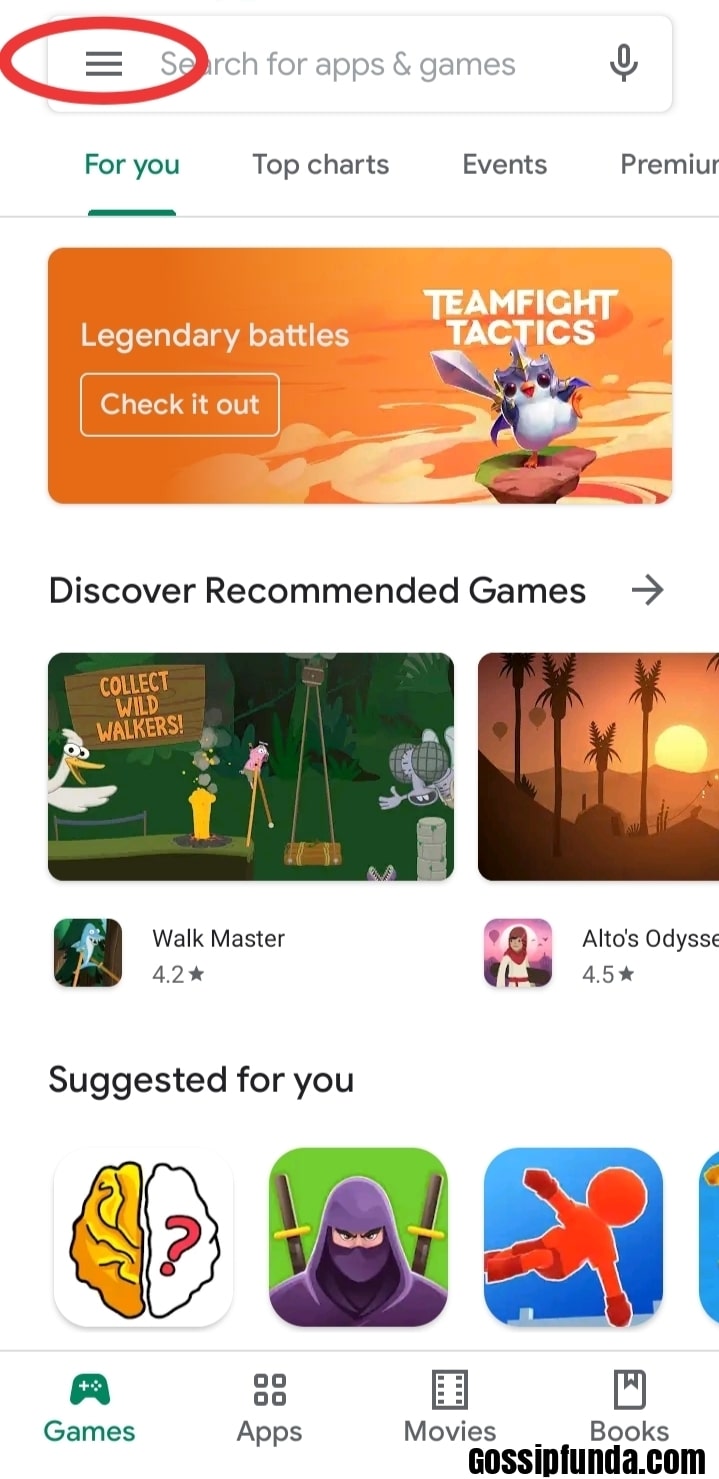A detailed screenshot from the Google Play Store displays a user browsing for apps and games. At the top of the screen, there's a highlighted hamburger menu, indicated by a red circle. This screenshot features several watermarks, including a large one that is gray and downward-facing with text that is difficult to read, potentially reading "tomorrow" or similar. Additionally, there are smaller, lighter watermarks angled to the right that read "GossipFunda.com." An overlay logo of GossipFunda is located in the bottom right corner.

In the primary search bar at the top, users can see options to search for apps and games, as well as a microphone icon for voice search. Various tabs are available for navigation, including "For You," "Top Charts," "Events," and "Premium," with "For You" being highlighted in green text with an underline.

Immediately beneath this, a wide promotional tile advertises "Legendary Battles, Teamfight Tactics," featuring an image of a small purple penguin wielding a sword against an orange background. Below this promotion, under the heading "Discover Recommended Games," there is a tile for the game "Walkmaster," showcasing what appears to be a bird on stilts with the tagline "Collect Wild Walkers." Beside this, a graphic of a sunset with palm trees is shown, even though the name of its associated item isn't visible. Below this image, the text "Alto's Odyssey" appears along with an icon of a person in a tunic, boasting a 4.5 rating.

Further down under "Walkmaster," a tree and fish graphic is displayed with a 4.2 rating next to the game "Alto." In the section "Suggested For You," images include a brain and a figure resembling a parkour warrior. An additional watermark on the image claims, "This image is protected."

At the bottom of the screenshot, tabs for "Games," "Apps," "Movies," and "Books" are visible, each accompanied by their respective icons. The "Games" section is highlighted in green with a game controller icon above it, indicating the current selection.